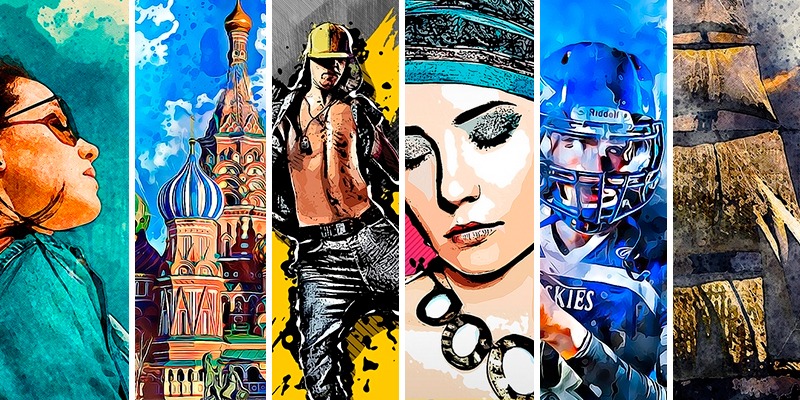The contemporary landscape-format image features six vibrant and vertically arranged illustrations, each separated by a thin white line to create distinct yet unified compositions.

Starting from the left:

1. **Woman with Sunglasses**: A striking illustration of a woman clad in a green top, looking upward towards the sun. She sports sunglasses and lipstick, set against a green background. Her expression and the upward gaze enhance the sense of contemplation.

2. **Colorful Russian Buildings**: The next vertical strip showcases an assembly of fantastical buildings reminiscent of Russian architecture, characterized by their vivid blues, reds, and greens. The buildings have rounded, Hershey Kiss-shaped domes, and each one features unique color patterns against a blue sky backdrop.

3. **Rapper with Baseball Hat**: This panel depicts a man in a dynamic stance, possibly mid-dance. He wears a yellow baseball cap, a necklace, and has tattoos on his bare chest, visible through an open black shirt. His yellow background accentuates the vibrancy of his presence.

4. **Woman with Eyes Closed**: An illustration of a woman with her eyes gently closed, adorned with glittery black eyeshadow and dark eyebrows. She wears a prominent large necklace and a sash across her head, further highlighted by her red lipstick. Her serene expression and contemporary look are set against a simple background.

5. **Football Player**: This image features a football player in a bright blue helmet and a matching blue and white jersey. The player's stance and the sense of motion, with his hand in view, suggest an active pose against a blue background.

6. **Abstract Black and Gold Forms**: The final panel is an abstract image with black and gold sections creating a mysterious and almost sail-like formation. These shapes cast subtle shadows, adding depth and intrigue to the composition.

All panels are unified by their modern, highly detailed, and colorful illustrative style, giving the overall image a cohesive and contemporary aesthetic.